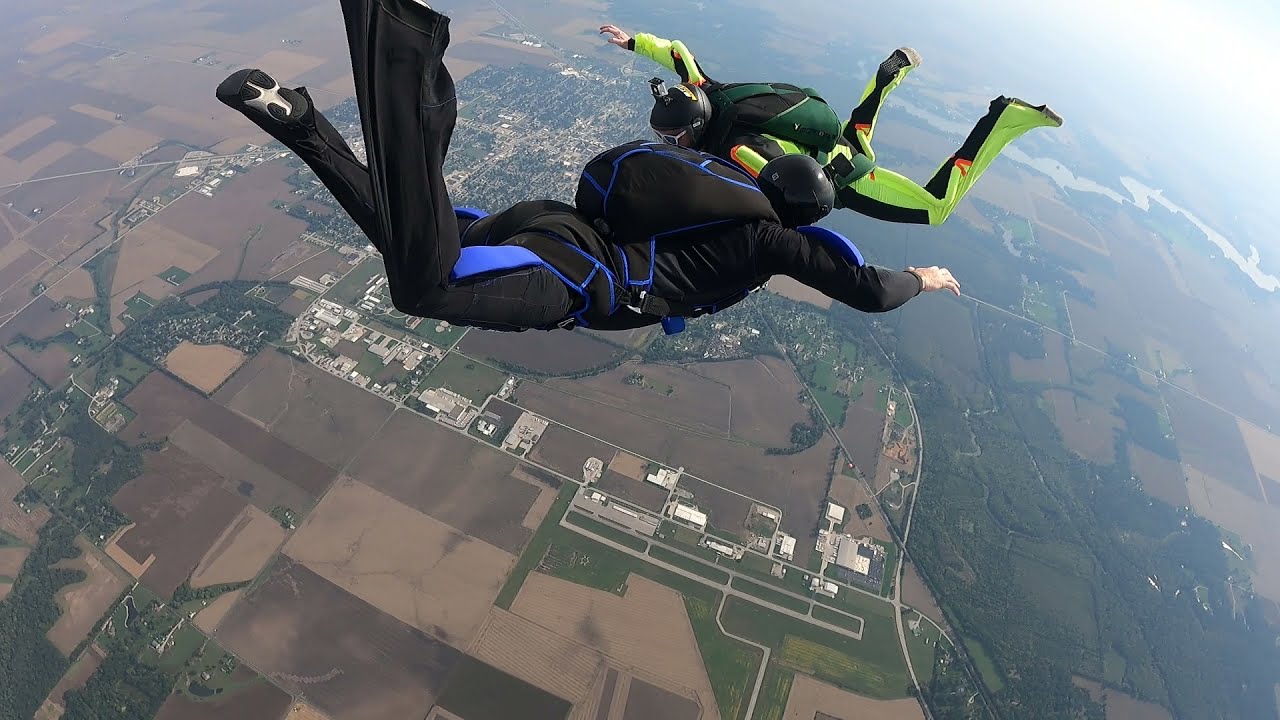This photograph captures a thrilling moment of two skydivers in midair. The duo appears to be holding hands as they float horizontally with their stomachs facing the ground far below. The skydiver closest to the camera sports a black skydiving suit accented with blue and wears a matching black helmet. His parachute bag, also designed in black with blue accents, rests securely on his back. His position has him facing to the right with his feet pointing to the left. The second skydiver, positioned slightly further and oriented in the opposite direction—head to the left and feet to the right—wears a vibrant neon yellowish-green jumpsuit with a contrasting green and black parachute bag. Both skydivers seem to have cameras attached to their helmets, possibly documenting their fall. Spread out beneath them is a stunning bird's-eye view of the earth, featuring a vast patchwork of green and brown fields, interspersed with small houses and buildings. A river is visible winding its way through the landscape, and a populated town sits northward, enhancing the scenic panorama from their lofty vantage point.